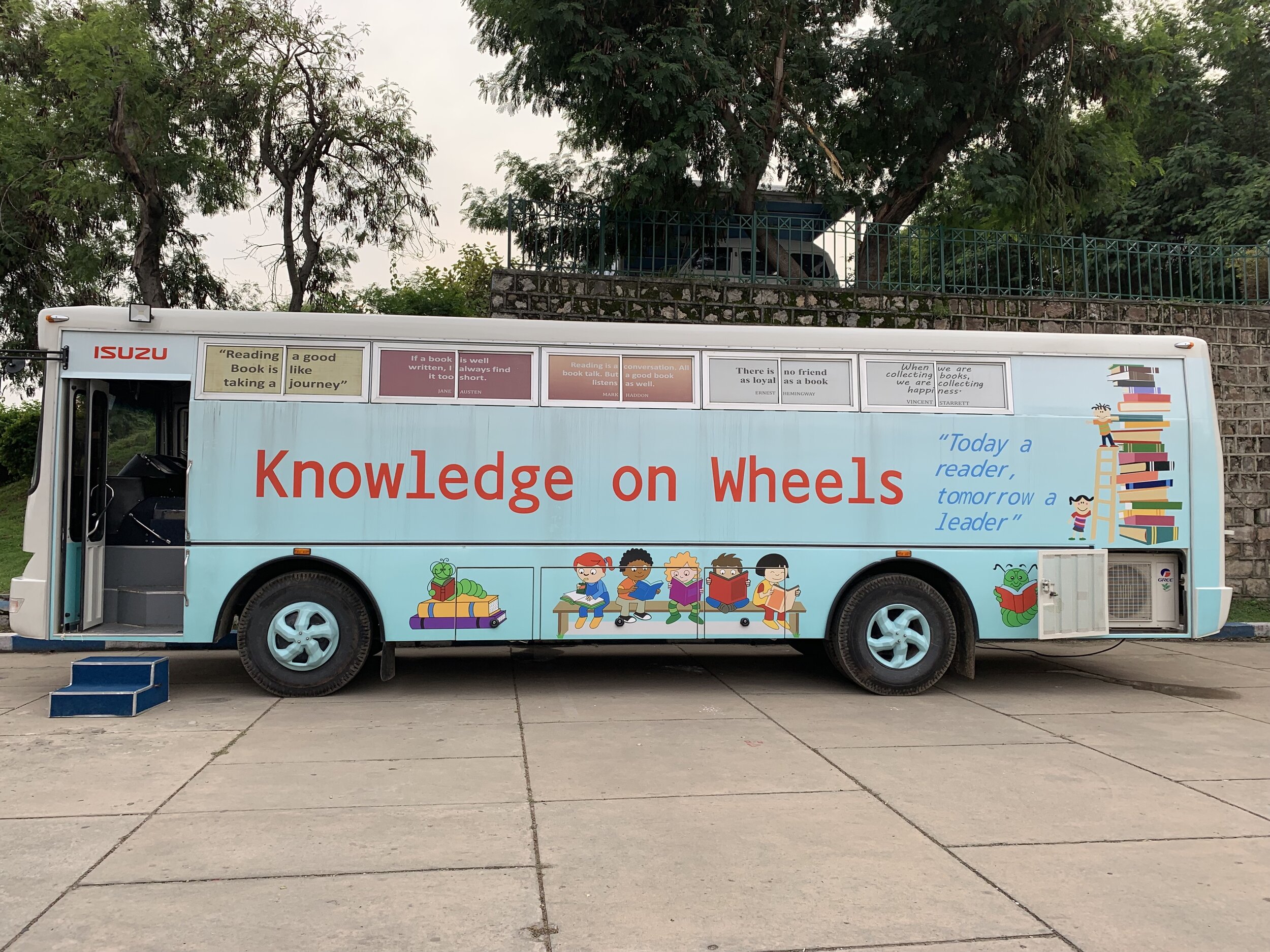This photo depicts a pale blue, customized school bus that has been transformed into a vibrant mobile library, possibly in Japan. The bus is situated on a concrete driveway, backed by a tall brick wall topped with a black gate, with trees visible in the background. Bold red text on the side of the bus proclaims "Knowledge on Wheels," alongside a slogan in blue that reads, "Today a Reader, Tomorrow a Leader." The bus is adorned with colorful illustrations, including a green bookworm sitting on a stack of books, five children reading on a bench, and another mural showing kids climbing a ladder up a towering stack of books. Above the bus door, which is open and flanked by a small blue step for easier access, there is red "Isuzu" text. Additionally, the bus features an air conditioning unit at the bottom corner beneath it, making it a cozy and inviting mobile learning center for children to explore the joy of reading.